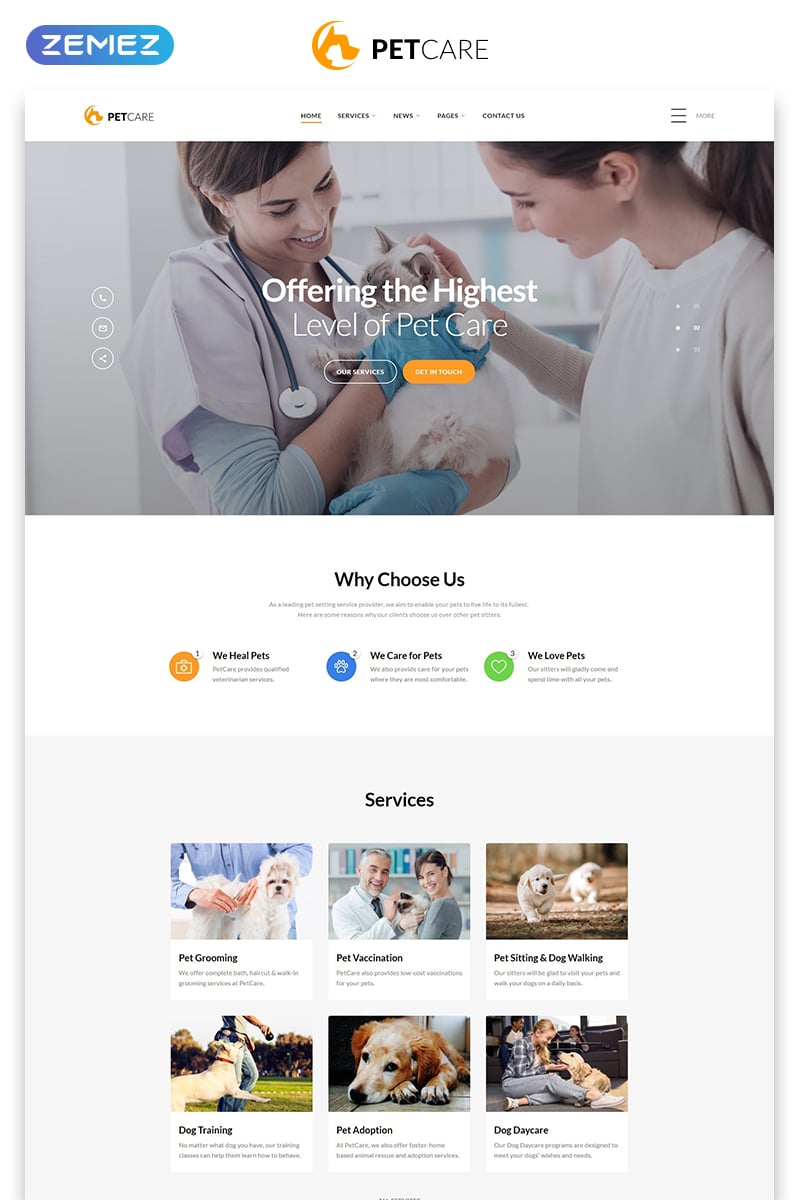This image is a detailed screenshot of a webpage dedicated to pet care services. The webpage has a clean white background at the top, prominently displaying the text "Pet Care" alongside an orange icon featuring a dog facing right and a cat facing left. In the top left corner, there is a blue oval shape with the text "ZEMEZ" inside it.

Below this, the navigation bar includes the same "Pet Care" text and icon on the left, followed by menu options: Home, Services, News, Pages, Contact Us, and a "More" menu on the right.

The main section of the page showcases a stock image of two women petting a cat in what appears to be a veterinary office. The woman on the left seems to be a veterinarian, as indicated by the stethoscope around her neck. She has brown hair tied up, is smiling while looking down at the cat, and is wearing a white uniform with blue gloves. The woman on the right, who is petting the cat, is clad in a long-sleeved white shirt and also has her hair tied back. The cat they are attending to is white.

Below the image, the section "Why Choose Us?" is introduced, with some descriptive text underneath, followed by three main options listed from left to right: "We Heal Pets," "We Care for Pets," and "We Love Pets." The bottom section of the webpage highlights various services, with the final service being "Dog Daycare."